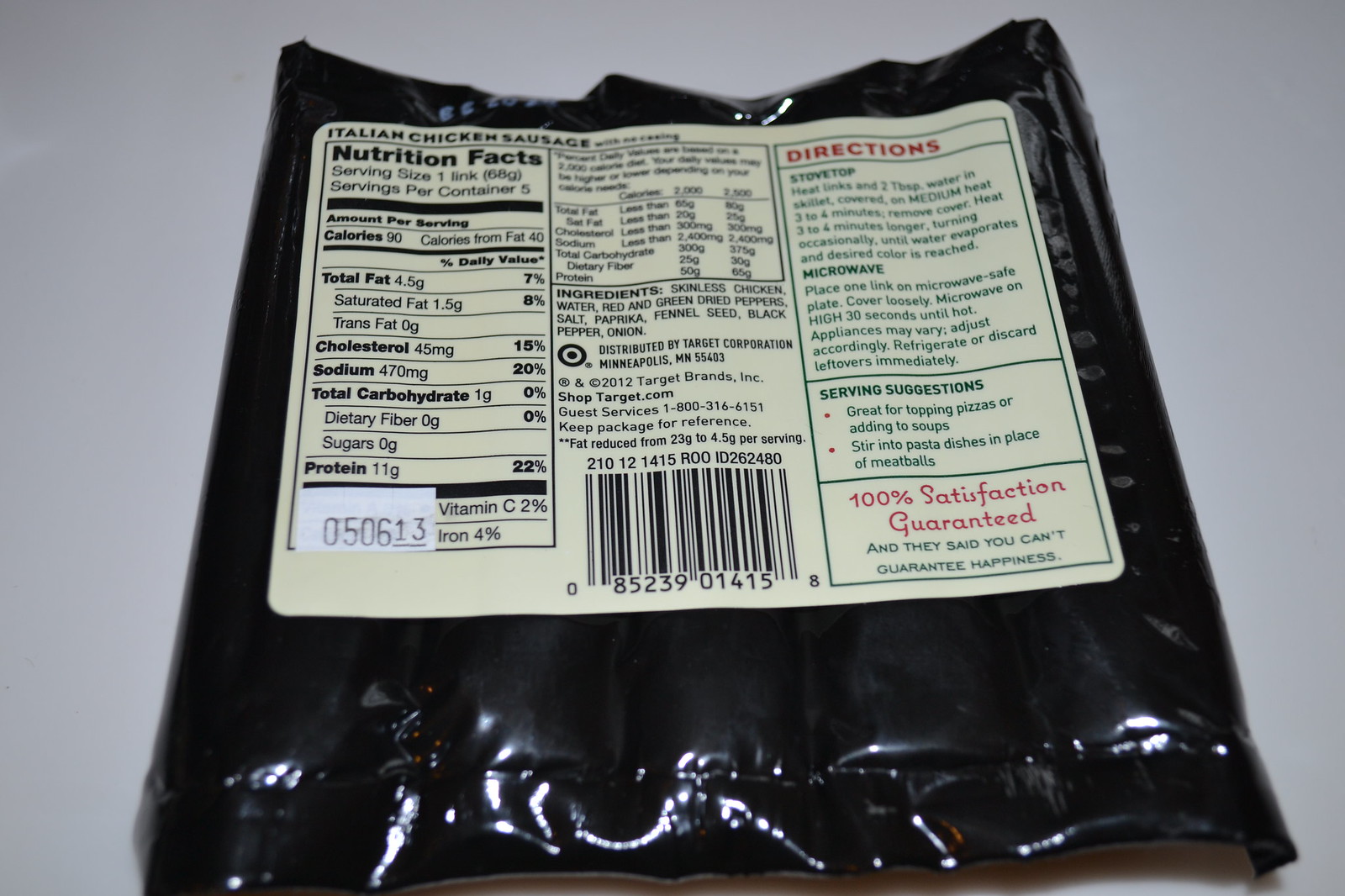Photographed against a pristine white tabletop background, a sleek black food package prominently displays its contents. The package, adorned with a vibrant yellow label, clearly identifies the product as "Italian Chicken Sausage." This enticing label is meticulously detailed, providing comprehensive nutritional information: each serving (one link) contains 90 calories (40 from fat), 4.5 grams of total fat (7% DV), 1.5 grams of saturated fat (8% DV), 0 grams of trans fat, 45 milligrams of cholesterol (15% DV), 470 milligrams of sodium (20% DV), 1 gram of total carbohydrates (0% DV), 0 grams of dietary fiber, 0 grams of sugar, and a substantial 11 grams of protein (22% DV).

The packaging includes a clear date code of "05-06-13" and proudly features the Target brand logo, indicating the product is distributed by Target Corporation, Minneapolis, Minnesota. The label directs consumers to shop at Target.com and reassures them with a "100% Satisfaction Guaranteed" promise.

For culinary inspiration, the packaging suggests versatile serving ideas: these savory sausages make an excellent topping for pizza, a hearty addition to soups, or a flavorful substitute for meatballs in pasta dishes. This detailed label ensures that consumers are not only informed about the product's nutritional benefits but also inspired to incorporate it creatively into their meals.